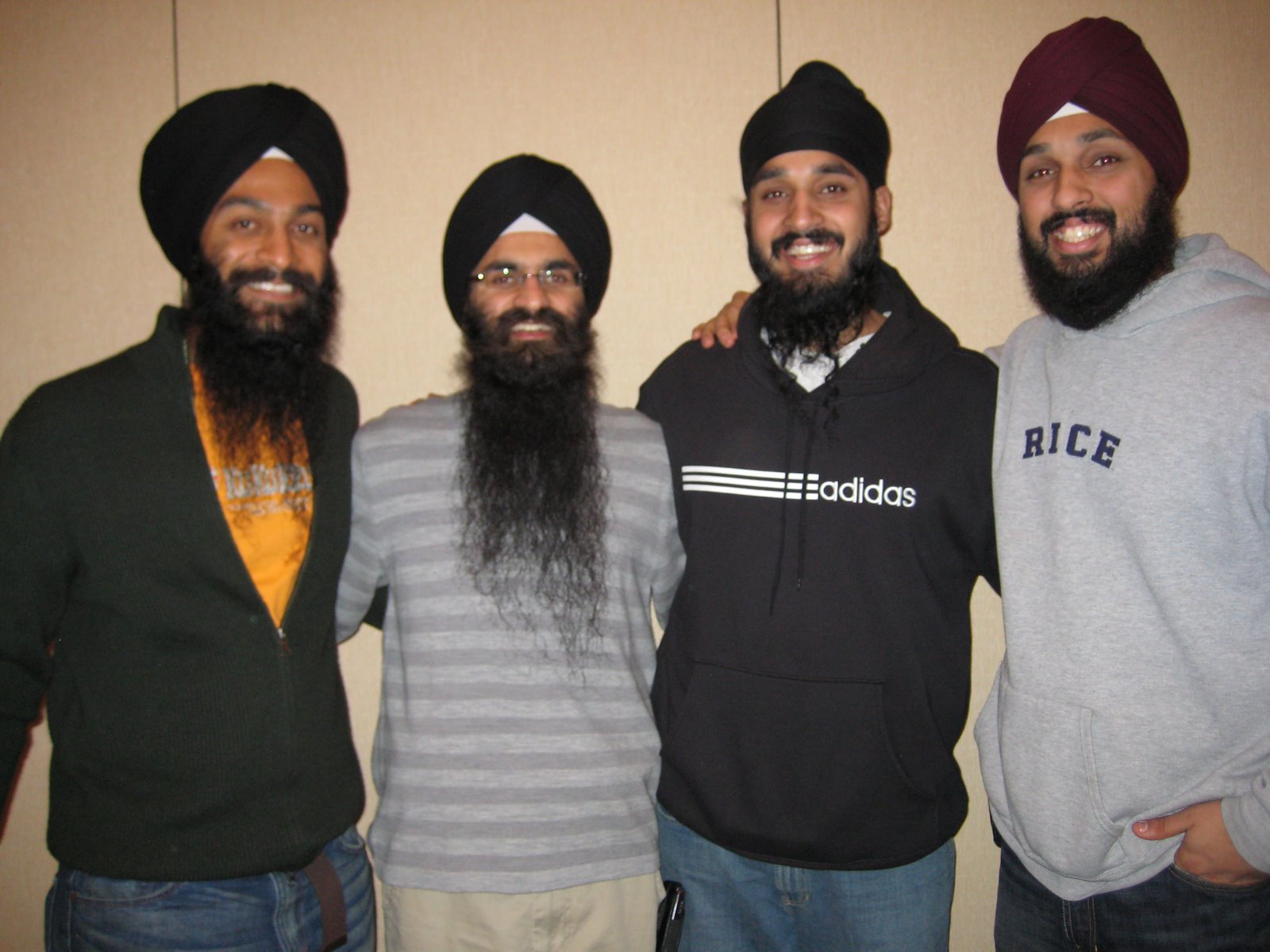This photograph features four Sikh men standing side by side, all donning black turbans and showcasing their long, black beards and mustaches. Each is smiling broadly, their happiness palpable. They are standing against a light, cream-colored paneled wall, seemingly inside a room.

Starting from the left, the first gentleman is wearing an orange t-shirt under an unzipped black sweatshirt. The second man, appearing shorter and older with the longest, wavy beard that reaches the middle of his stomach, is dressed in a light gray and dark gray striped t-shirt and khaki pants. The third man is clad in a gray Adidas tracksuit with white stripes and blue jeans. The rightmost man, who has his hand in his pocket and his arm around the shoulder of the man next to him, is wearing a gray hoodie with the word "RICE" printed in dark blue letters, paired with grayish jeans.

Their black turbans mostly have a peak with some white cloth showing underneath, except for the third man's turban, which resembles a beanie. The men exhibit a unified appearance with their similar attire and expressions, creating a harmonious and joyful scene.